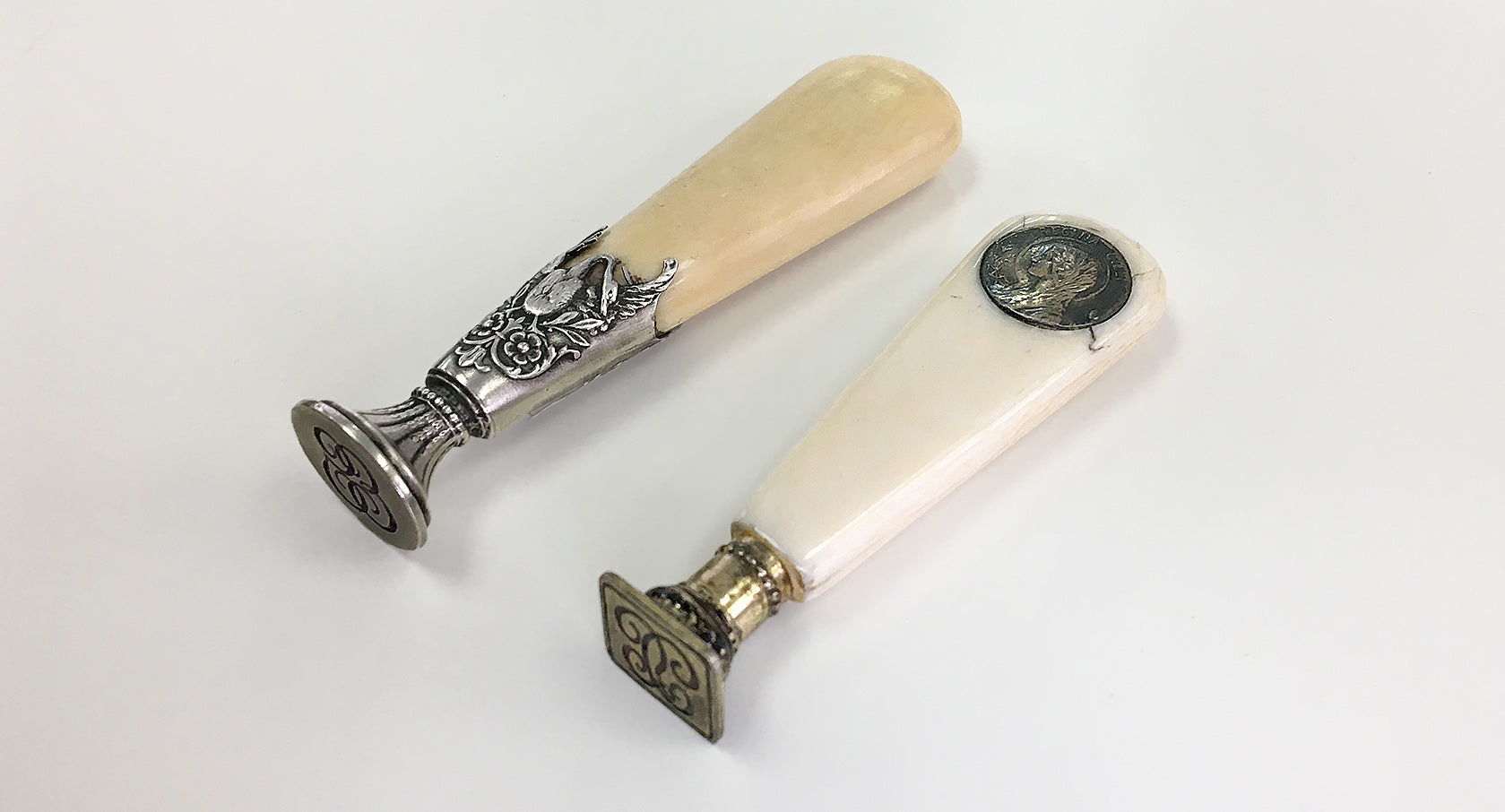The photo showcases two vintage, stamp-like tools positioned on a light gray surface. The tool on the top left has a beige wooden handle that transitions into a round silver base adorned with floral patterns. The tool on the bottom right features a marbled white handle leading to a square metal base with a golden, coin-like emblem displaying a woman's profile. Both tools are oriented with their handles pointing upwards and slightly to the left. Soft, dim shadows are cast from the lighting, enhancing the well-lit image's detailed and nostalgic aesthetic.